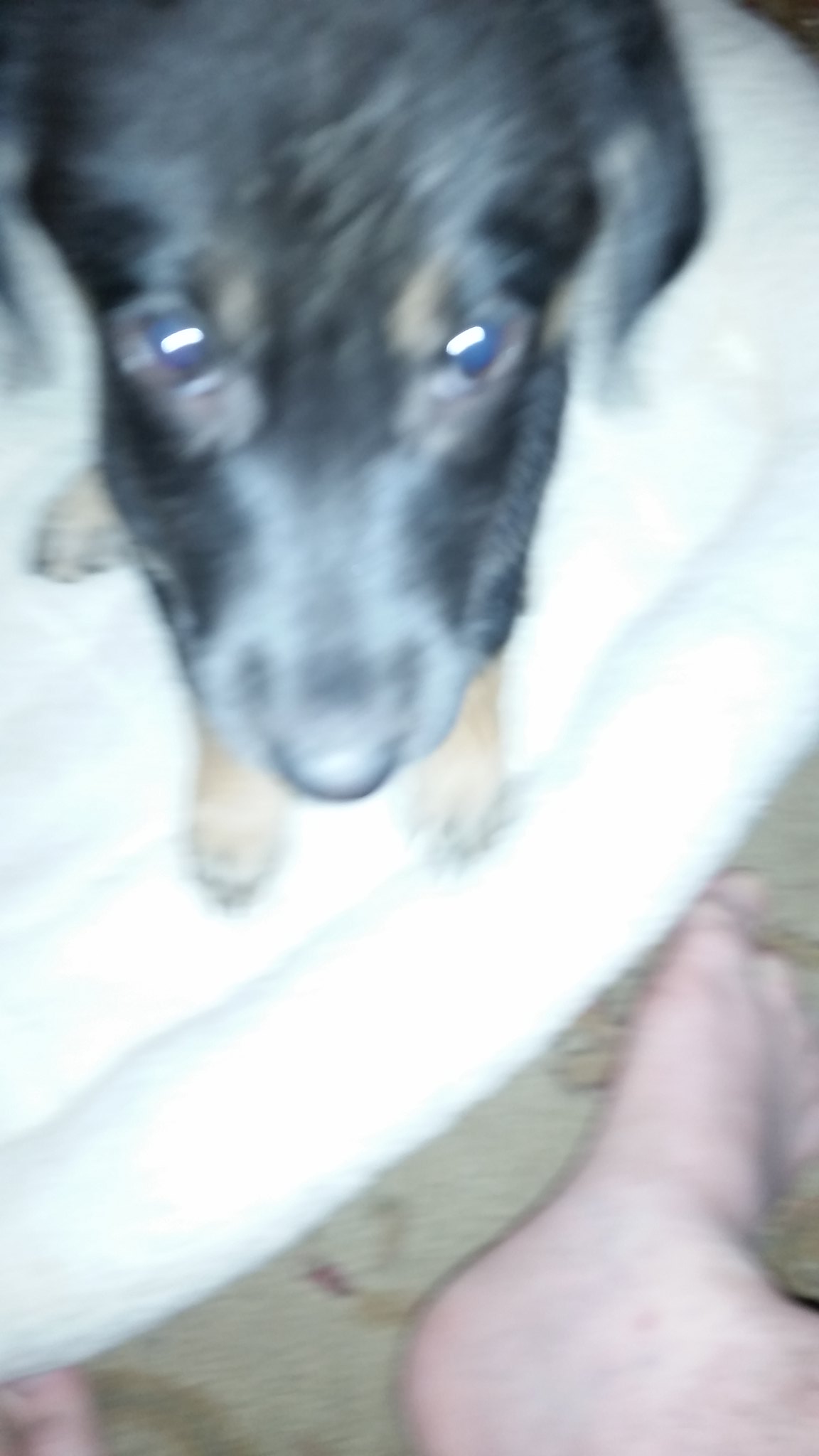This is a very blurry and slightly grainy photograph featuring a partial view of a person's bare feet with light skin, standing on a beige carpet. Centered in the image, laying on a light blue, fluffy dog bed, is a dog with a mostly black face and nose, adorned with grey around the eyes and ears. The dog's eyes are blue and reflect the light from the camera flash, which also gives its nose a slightly washed-out appearance. The dog, which has a black and tan coat with visible tan paws, displays an eager expression as it looks up at the camera. The image captures three of the dog’s paws and part of its legs.